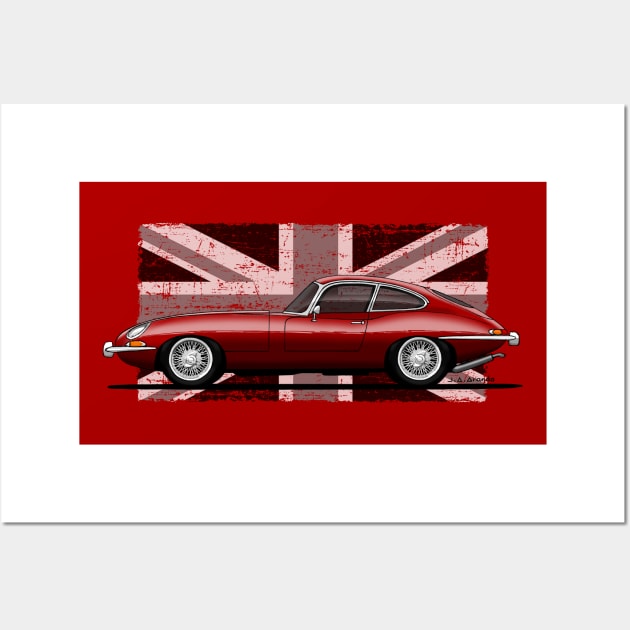This detailed image features a striking, fire-engine red vintage sports car, likely a Jaguar from the 1960s. The car boasts a sleek, aerodynamic design with a long hood and a compact, turtle-shaped rooftop. It’s a two-door model, showcasing black wheels and silver trim that accentuates its shiny red body. This car is positioned side-on, facing to the left, and sits in front of a vintage British flag rendered in a monotone red hue, contributing to the image's dramatic aesthetic. The composition is framed by a thick red border against a white paper-like background, with a faint gray backdrop further highlighting the central elements. There is also subtle black text located in the bottom right corner, which appears to be an author's name, "J.A. Andrus." The artistic nature of the image, possibly a painting or illustration, is underscored by the striking combination of colors and the faded, worn look of the flag.